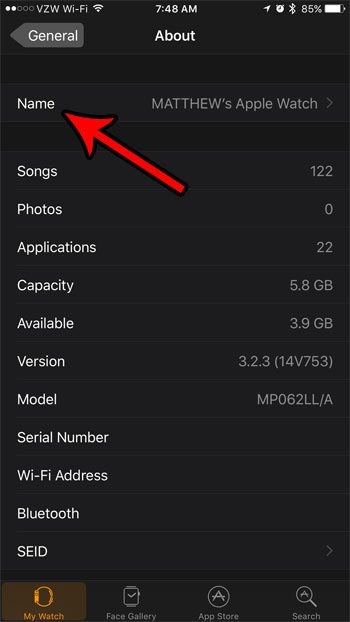The image depicts a screenshot of an Apple Watch interface. The background is a black rectangle with several informational elements displayed. 

On the top-left corner, there are five small dots; two are filled in with white, while the remaining three are outlined in white. Just below these dots, the text "VZW" is displayed, followed by the Wi-Fi symbol and the text "Wi-Fi." 

Centrally located is the time "7:48 AM," accompanied by a slightly tilted 'M' symbol, an icon of an alarm clock, and two triangles pointing right with a partial third one underneath, representing the alarm or timer. To the right of these, the battery icon indicates that the battery is at 85% capacity.

Underneath this, the word “Name” is written in white text with a red arrow outlined in black pointing towards it. Following this, the text "Matthews Apple Watch" appears with an arrow pointing to the right. Additional details such as "Songs, Photos, Application, Capacity, Available, Verizon Model, Version, Model, Serial Number, Wi-Fi access, Bluetooth, SEID" are listed below. On the right-hand side, numerical values "12/20/22, 5.8 GB, 3.9 GB, 3.2.3 (14V753), MP062LL-A" are provided.

There is a partially transparent yellow rectangle overlaying the background, containing what seems to be an image or icon of a bracelet or watch with the label "My Watch." Below this, there is a gray rectangle with a checkmark inside it, labeled "Face Gallery." Further down, there is a white-outlined circle with a capital 'A' inside it, indicating the "App Store." Lastly, there is a white-outlined magnifying glass icon with something in the middle labeled as "Search."